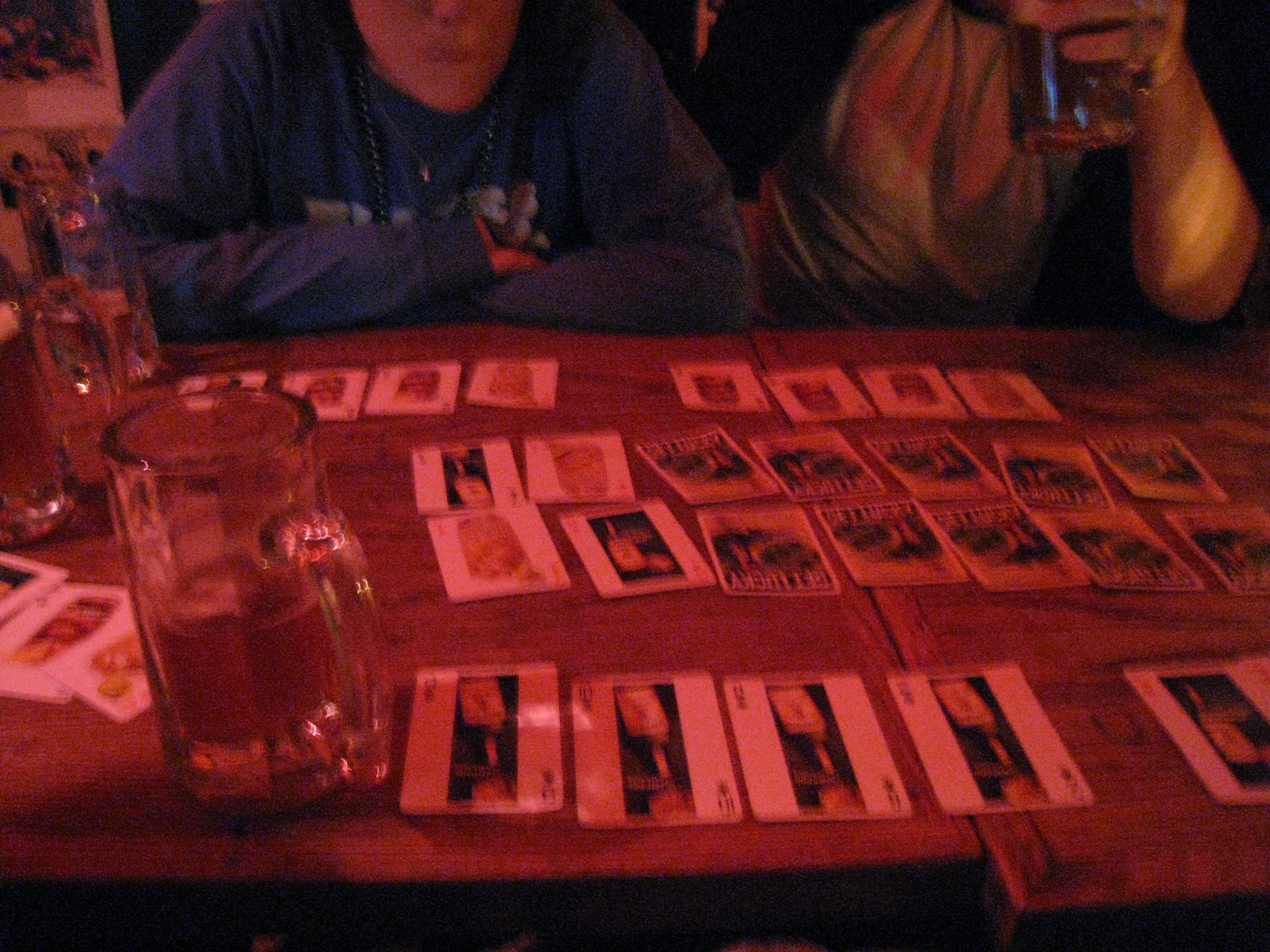In an atmospheric indoor setting captured at night, a striking red glow envelops the photograph, casting an enigmatic hue over the scene. The image focuses on two slightly misaligned wooden tables, hinting at an impromptu gathering. In the bottom left corner, a large glass stein half-filled with beer stands as a testament to the photographer's vantage point.

Across the table, two men are engaged in what appears to be a casual, yet intriguing activity. On the top left, a man wearing a dark blue sweatshirt with a largely obscured design sits with his arms crossed. A beer mug rests beside him to his right. Opposite him, in the top right corner, another man sports a two-tone short-sleeve shirt, with grey and dark-colored sleeves. He holds his beer glass firmly in his left hand.

The table is scattered with various cards that feature images of alcohol and booze bottles, suggesting a specialized card game or collection, possibly distributed by the bar. The low light and the red tint add a layer of mystery and camaraderie to the entire scene.